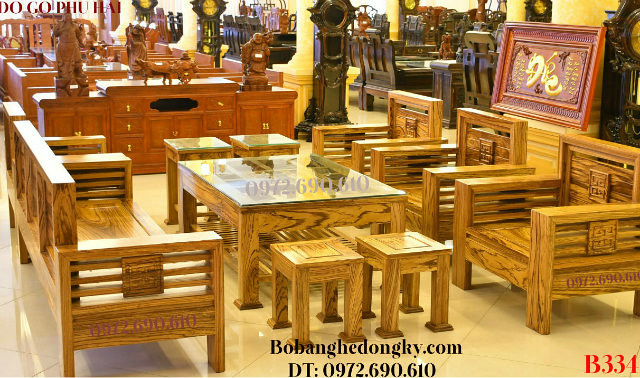The image depicts an Asian-inspired furniture store, showcasing a variety of finely crafted wooden furniture. Central to the scene is a sturdy wooden bench positioned in front of a large wooden table with a glass surface, flanked by three distinctly square wooden chairs. This table is accompanied by four end tables, two on each side. The store also features an elegant, long buffet table made from thick brown wood adorned with gold hardware. Surrounding the central display are various other wooden pieces, including hand-carved statues and classical-style floor clocks resembling grandfather clocks. Text at the bottom reads "bobanghedongky.com" alongside numerical codes, including "DT0972.690.610" and "B334" in bold red in the lower right corner, hinting at the store's international and possibly non-English background.